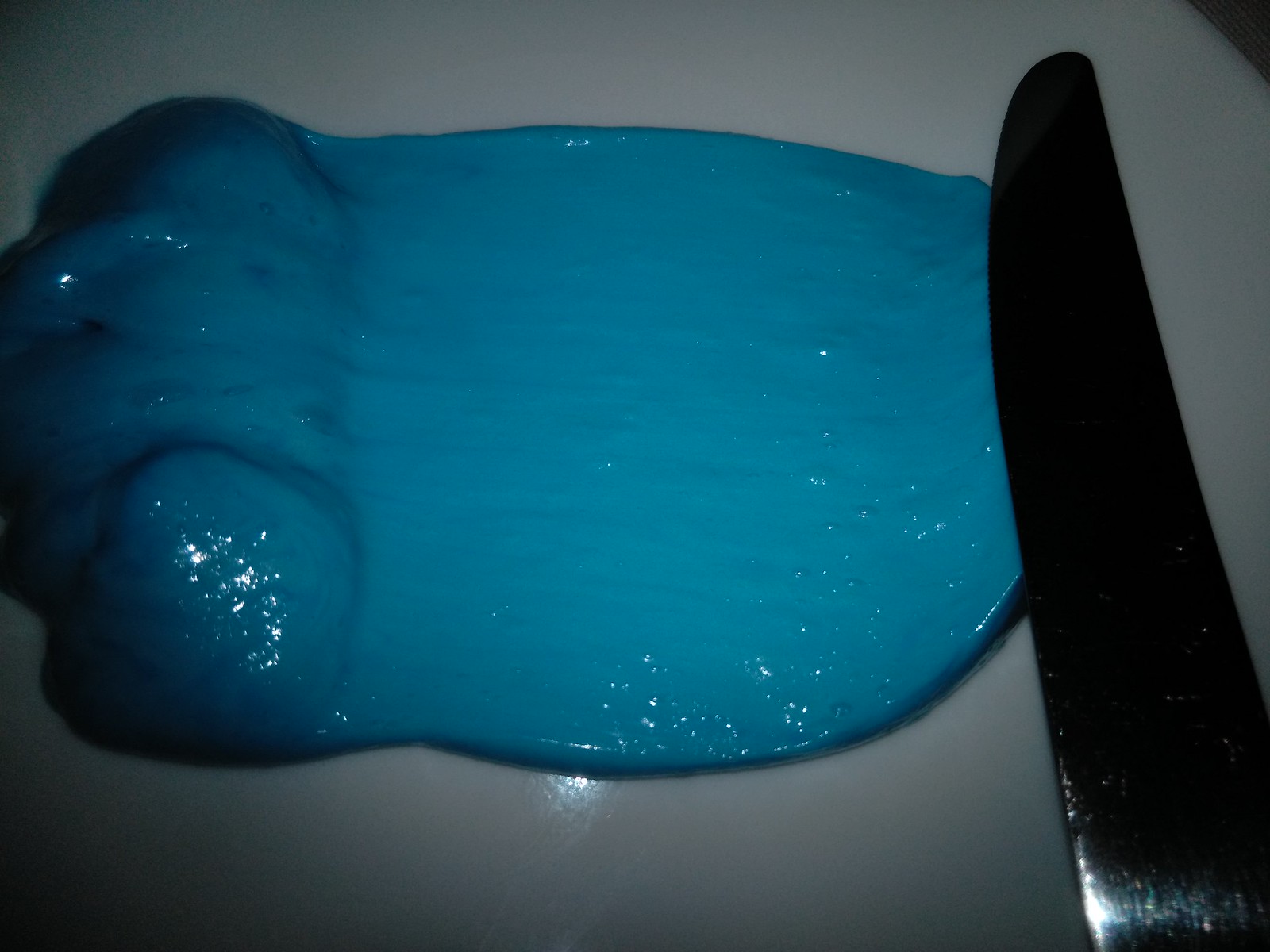This photo captures a close-up image of a silver butter knife poised over a white surface, likely a plate. The knife appears to have recently spread a dense, shiny blue substance that exhibits a wet, gel-like consistency. The gooey material has a vivid blue hue, with light reflecting off its surface, accentuating its smooth yet slightly globular texture. Air bubbles are visible within the spread substance, lending to its bumpy appearance on the left side, while the right side of the blue material appears more evenly spread and smooth. The image is minimalistic, focusing solely on the interaction between the knife and the mysterious blue blob, creating a curious and visually intriguing scenario.